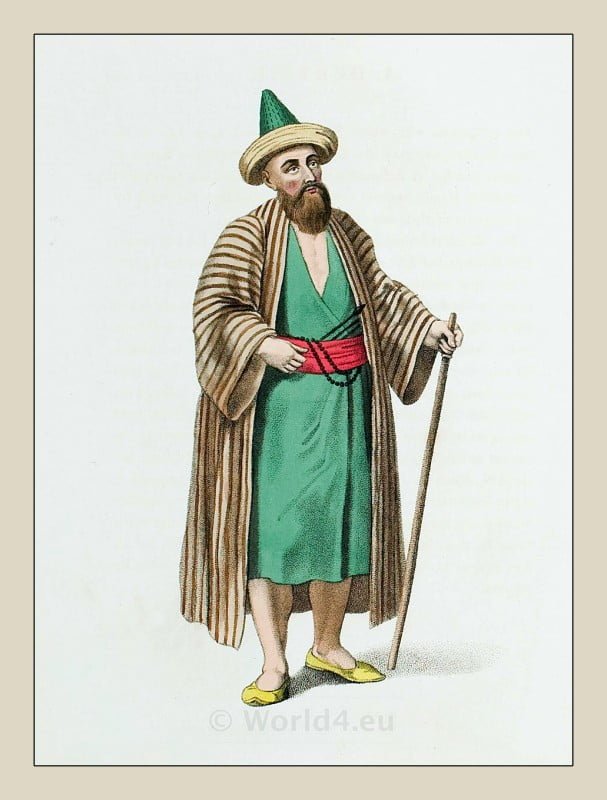The image features an illustration of a man standing centrally against a white background with a beige border. This man is clad in a distinctive outfit: a green gown cinched at the waist with a red sash adorned with black beads. Over this gown, he wears a long, brown robe characterized by dark brown horizontal stripes. His footwear consists of yellow slippers, and he accessorizes with a cone-shaped hat that is green with a beige brim. The man, who sports a long brown beard and rosy cheeks, is holding a thin walking stick in his right hand and appears to be looking upward. At the bottom of the picture, there is a text that reads “world4.eu” enclosed in a circle.